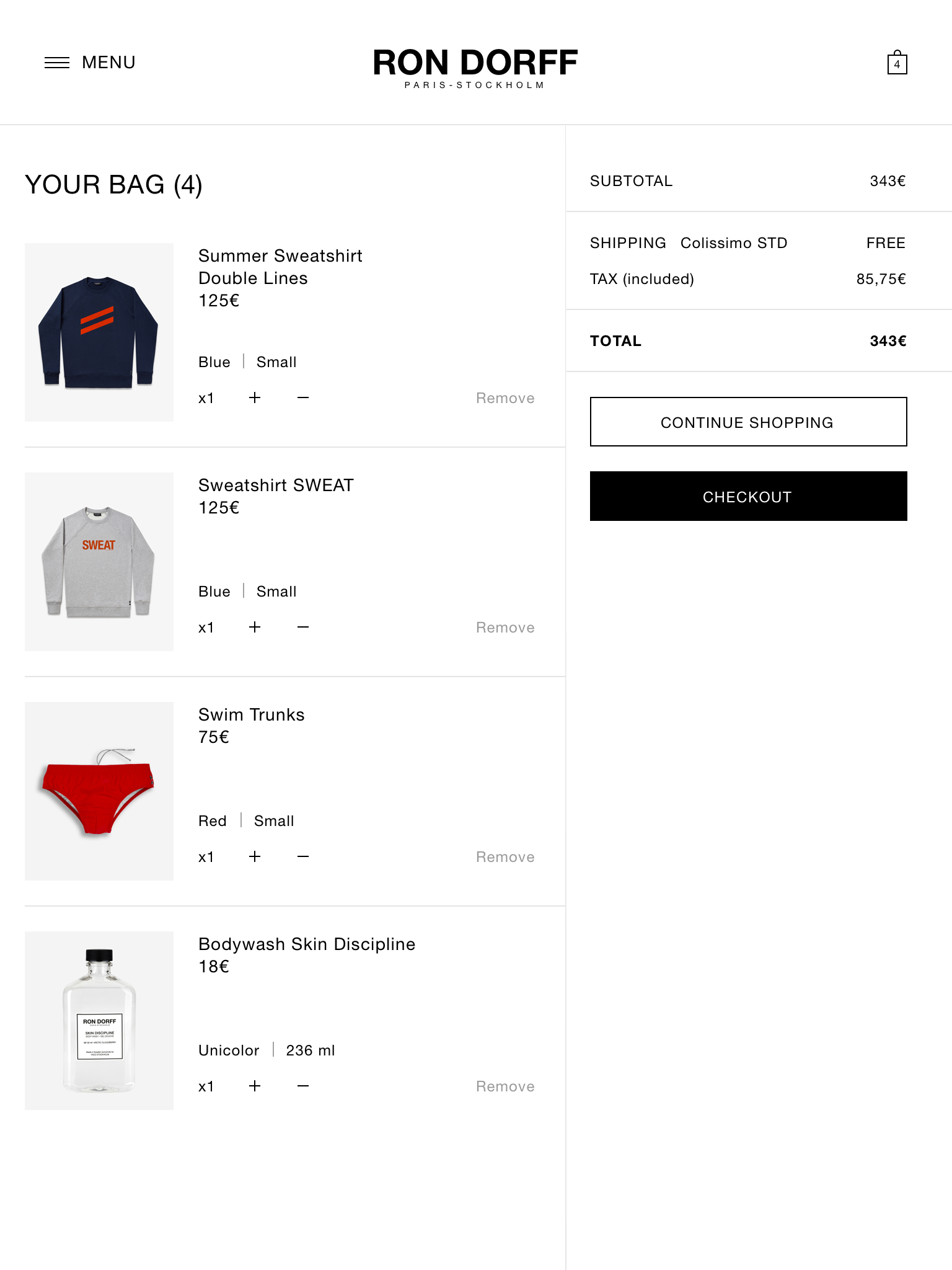Screenshot of an apparel website storefront, prominently displaying the brand "Rondorf" with the tagline "Paris-Stockholm." At the top left corner, there is a hamburger menu for easy navigation. The company name is centered at the top of the page, while the top right corner hosts a shopping bag icon indicating four items inside.

The screenshot specifically captures the shopping bag page, titled "Your Bag" with a detailed list of four items: a Summer Sweatshirt, a Double Lines Sweatshirt, a "Sweat" print sweatshirt, a pair of Swim Trunks, and a Body Wash. These items are neatly listed on the left side of the screen.

On the right side, the subtotal cost is displayed, totaling 343 euros. Beneath this, it mentions "Free Shipping" and a tax amount of 85.75 euros, summing to the same subtotal figure—343 euros, confirming that tax is included in the total.

Below the cost breakdown are two prominent buttons: one for "Continue Shopping" and another for proceeding to "Checkout."